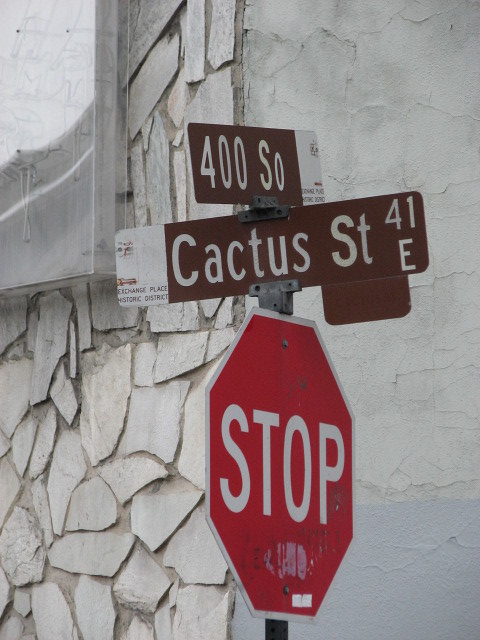The image features a prominently displayed red stop sign with the word "STOP" emblazoned in white. Above the stop sign are two intersecting street signs, arranged in a crisscross pattern, indicating different street names. The top street sign reads "400 SO" while the bottom sign states "Cactus Street 41 East"; both signs are brown with white text. These signs are securely attached to the top of the stop sign by a visible metal bracket. In the background of the image, a building is partially visible, constructed from a multitude of stones that combine to create a whitish-gray, concrete-like exterior.